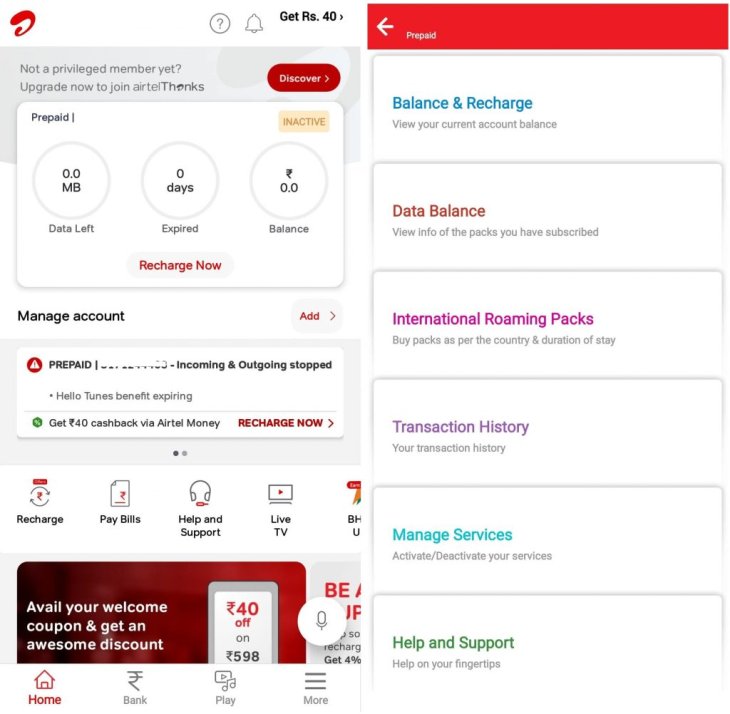This image is a screenshot of a mobile app interface, potentially related to a telecommunications or mobile services provider. It showcases two side-by-side screenshots, each depicting different sections of the app.

**Left Screenshot**:
- **Header**: Indicates usage summary with labels such as "0 MB of data left," "0 days," "Expired," "0 in balance," and "Prepaid is inactive."
- **Button**: A prominent "Recharge Now" button is visible.
- **Account Management Section**: Options to manage the user's account, such as "Add an Account" and another "Recharge Account" button. 
- **Menu Options with Icons**: Including "Recharge Account," "Pay Your Bills," "Help and Support," "Live TV."
- **Navigation Bar at the Bottom**: Displays four icons – "Home," "Bank," "Play," and "Menu."

**Right Screenshot**:
- **Section Label**: The section appears to be "Prepaid."
- **Tabs**: Various tabs available for the user to interact with, including "Balance and Recharge," "Data Balance," "International Roaming," "Packs," "Transaction History," "Manage Services," and "Help and Support."
- **Aesthetic Details**: Each tab is color-coded with hues such as blue, brown, purple, lilac, light blue, and green for ease of navigation and visual appeal.